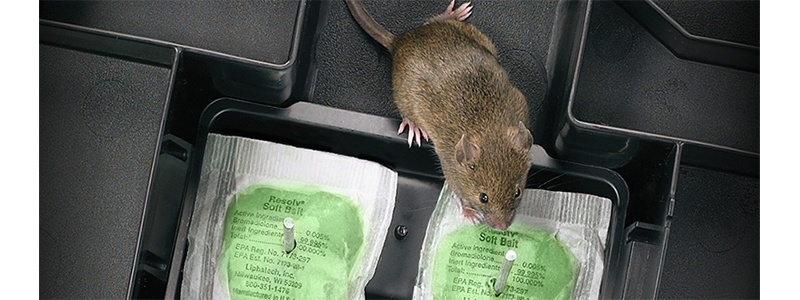The image taken from a top view shows a brown mouse with pink feet situated in a black compartmentalized area. In the center of the frame, the mouse is seen with one foot resting on one of two silver bags, which contain green bait material labeled "Resolve Soft Baits" in black text. The bags, located at the bottom of the image, have been punctured through with a metal rod.